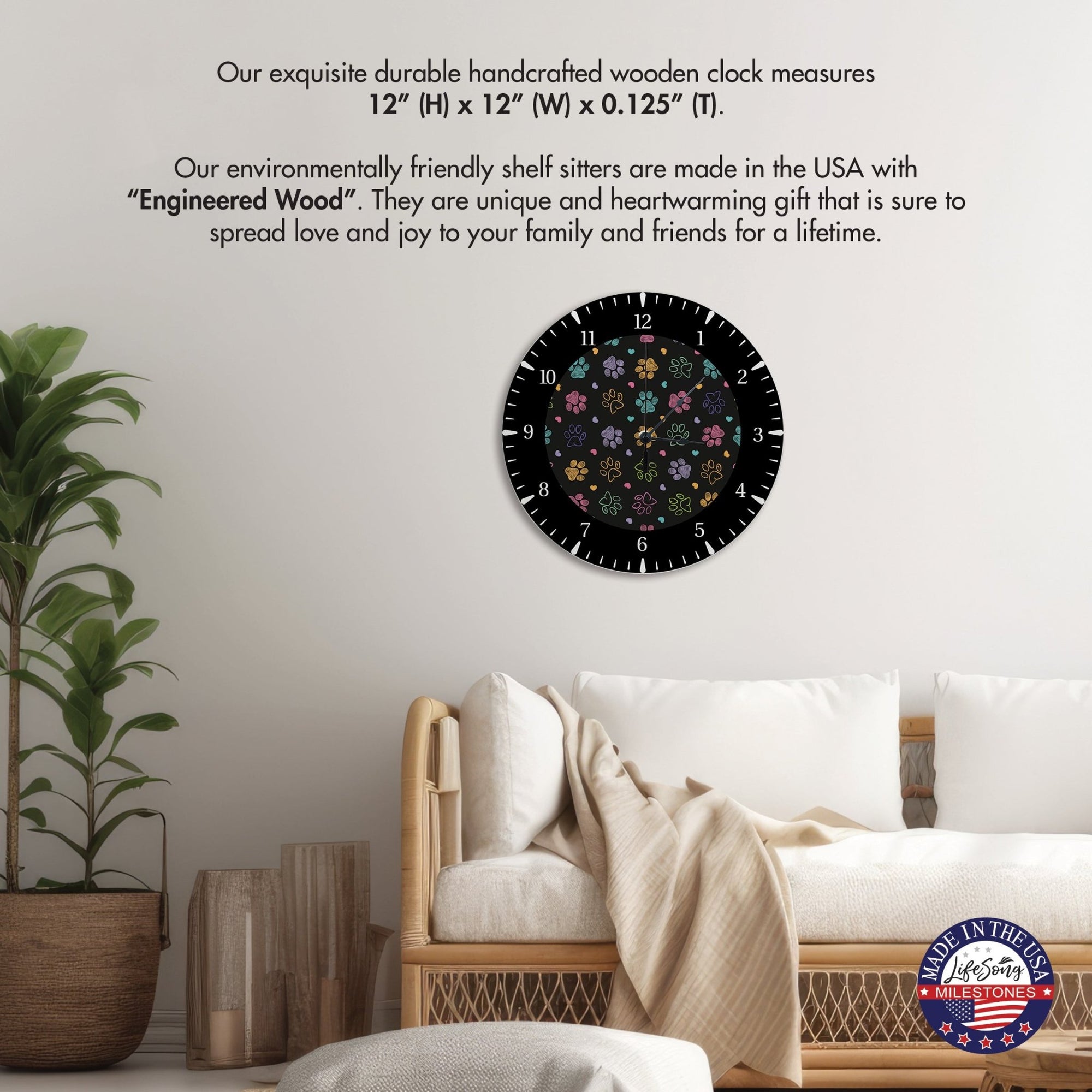The staged product photograph showcases a stylish, handcrafted black wooden clock mounted on a light gray wall, serving as a centerpiece in a tastefully decorated living room scene. The clock stands out with its white numbers and tick marks, alongside a vibrant and multicolored paw pattern in the circular center, consisting of hues like blue, red, yellow, green, and more. The clock features thin metal hour, minute, and second hands. 

Above the clock, black text highlights its distinct qualities: "Our exquisite, durable, handcrafted wooden clock measures 12 inches in height, 12 inches in width, and 0.125 inches in thickness. Our environmentally friendly shelf sitters are made in the USA with engineered wood. They're a unique and heartwarming gift that is sure to spread love and joy to your family and friends for a lifetime."

The room's design includes various elements that enhance the photograph's appeal: a white wicker couch with white cushions, a beige quilt, and a fallen pillow, adding a cozy touch. To the left of the clock, a tall indoor plant with large green leaves is placed in a brown vase, next to cylindrical items resembling lamps or candle stands. The logo situated at the bottom right corner of the image features a blue circle with the inscription "Made in the USA," including the words "Life Song Milestones" and five red stars along the bottom. 

This detailed setting and informative text beautifully combine to create an engaging and visually appealing advertisement for the clock.